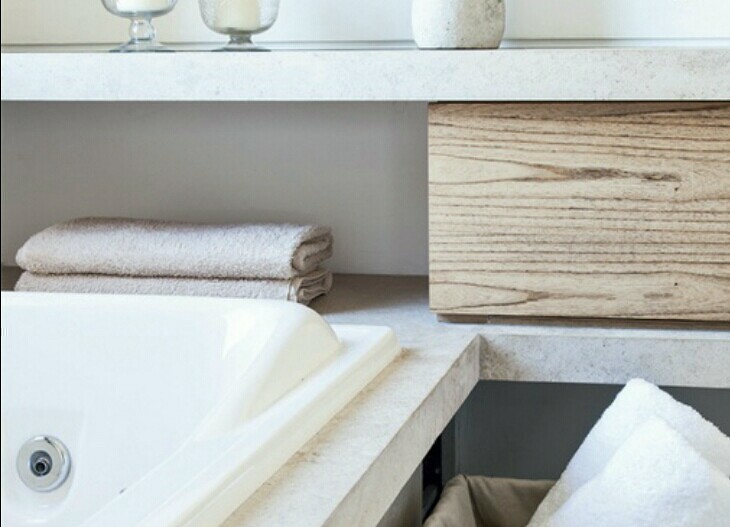The image captures a cozy bathroom setting, prominently featuring a white ceramic soaker tub situated to the left. The tub is equipped with a silver fixture, likely part of the pump system for water circulation. The back edge of the tub has an integrated white shelf adorned with a couple of neatly folded washcloths and a small wooden box. Above this shelf is another ledge showcasing a few items, including a clear pedestal glass and a shorter pedestal glass alongside a mysterious container.

To the right edge of the tub, a corner of what seems to be a brown-colored laundry hamper is visible, draped with cloth and containing a few folded white towels. Adjacent to this hamper is the door to a storage closet, likely situated under the tub, adding to the bathroom's functional yet stylish charm.